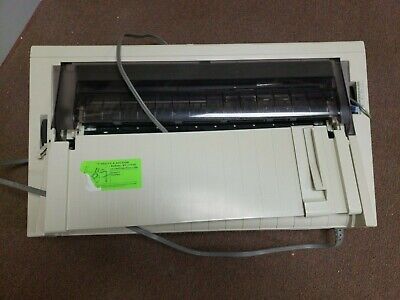The photograph depicts an old, seemingly non-functional dot matrix printer with an off-white colored housing. A grey power cable snakes from the back of the printer, looping under and through the device, ultimately emerging from the front. The top of the printer features a tilted paper tray that appears to be partially detached on one side. There's a transparent black rectangle serving as a viewport into the internals of the machine, where a black spool-like structure is visible. A green sticker can be seen on the right corner of the printer, though the text is unreadable. The device is situated on a surface that could be either a wooden table or brown carpet, with some grey area visible in the background, possibly a wall or flooring.